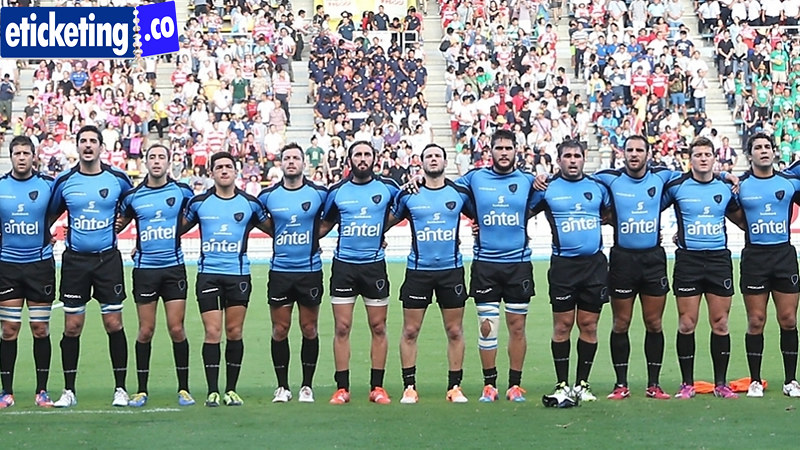This is a detailed photograph of a European football, also known as soccer, team standing arm in arm on a field in a large stadium. The team consists of 12 players dressed in blue jerseys with "A-N-T-E-L" written on the chest, black shorts, and black socks. They are wearing a variety of brightly colored soccer cleats, including shades of pink, white, blue, green, red, orange, and purple. The players are standing shoulder to shoulder, gazing slightly above the camera, possibly during a national anthem. The background reveals a well-maintained, lush green field and spectator-filled stands, with an area of fans in coordinated black or dark blue outfits on the left side, potentially a cheer group. The upper left corner of the image displays the text "eTicketing.co," adding to the professional atmosphere of the scene.